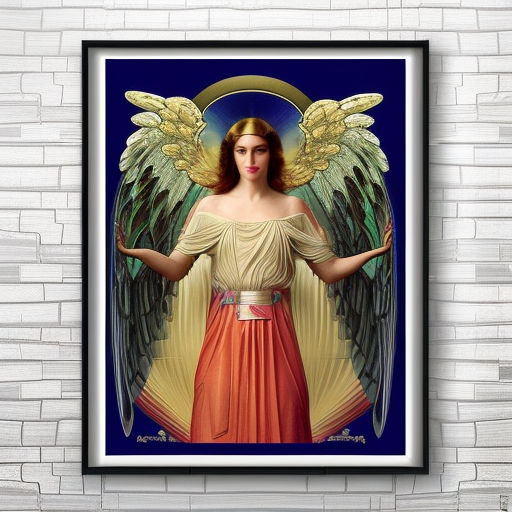The image showcases a detailed painting of a female angel set against a textured white and gray brick wall. The angel is depicted against a dark blue background and is framed with a white and black border. She has long, somewhat red hair and wears a golden cowl. Her attire consists of a flowing gown in shades of yellow, red, and light cream, fastened with a belt at her waist. She holds her hands outstretched at shoulder height. Her majestic wings feature a striking blend of green, dark blue, teal, and gold hues. Adding an ethereal touch, she also appears to have a half-halo behind her head.